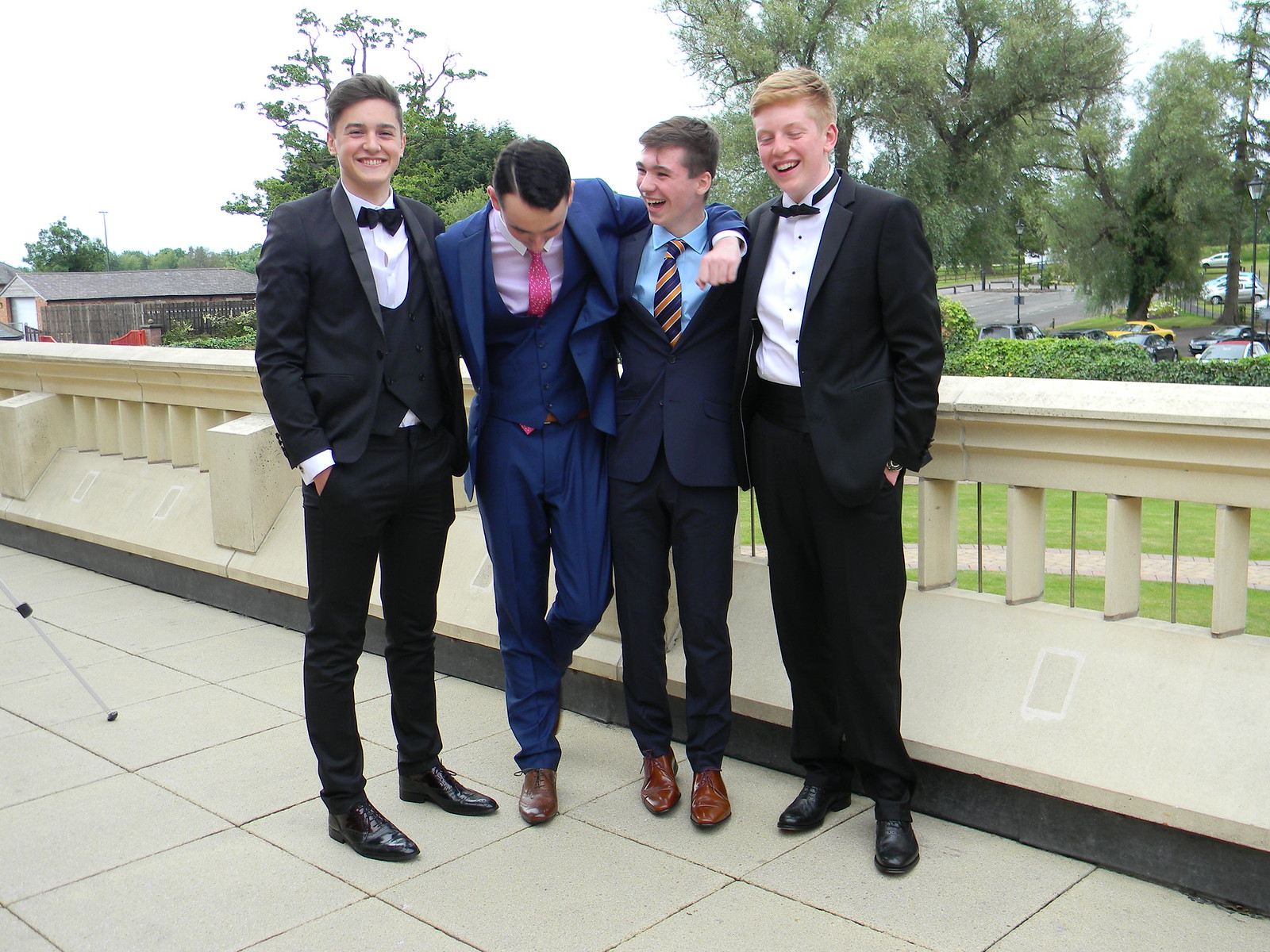In this rectangular daytime color photograph, four young Caucasian men with short haircuts stand side by side, their arms around each other, all smiling warmly. Each is sharply dressed: the young man on the left dons a black tuxedo with a black bow tie and white shirt, looking directly at the camera. The second young man wears a blue tuxedo with a pink shirt and tie, his head bent down, revealing his short brown hair as he smiles. His left arm wraps around the neck of the third young man, who is clad in a navy blue tuxedo with a blue shirt and a striped blue and orange tie. This young man glances towards his friend, smiling and laughing. The fourth young man on the right, with blondish-red hair, wears a black tuxedo paired with a black bow tie and white shirt, his eyes closed as he smiles. The group stands on white towels in front of what appears to be white columns, with a stone patio beneath their feet. Behind them, lush green trees, a yellow car, and a black car are visible, indicating a parking lot filled with more vehicles beyond the scene.